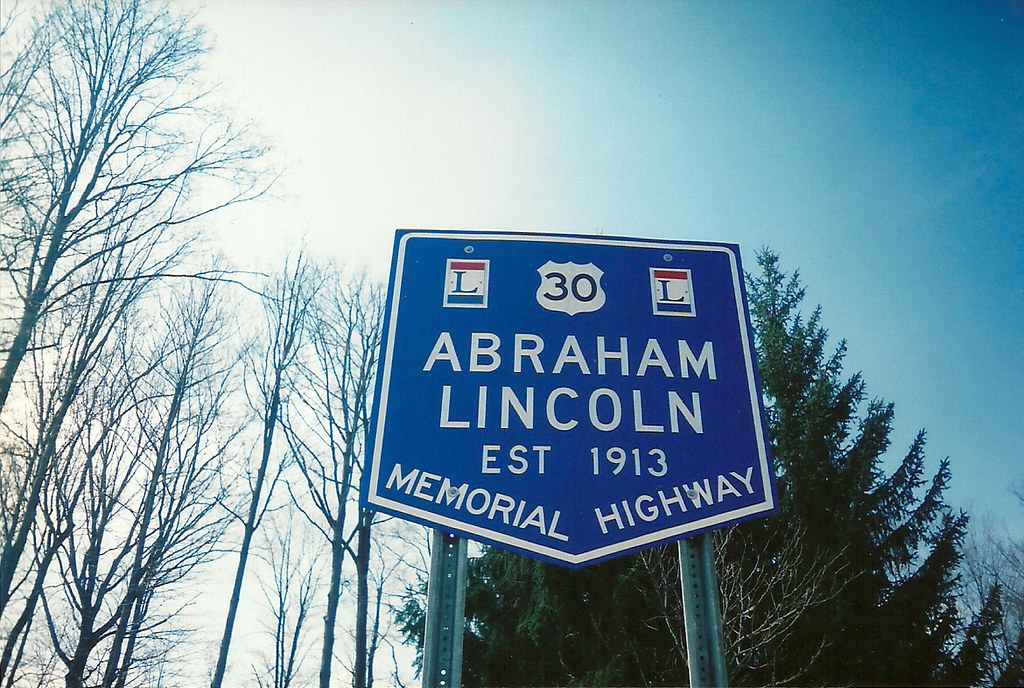A weathered sign marking the Abraham Lincoln Memorial Highway stands prominently amidst a scenic backdrop of diverse trees. On the left, barren trees, likely oak or maple, exhibit the stark beauty of winter, their branches stripped of leaves. To the right, resilient pine trees retain their green needles, a characteristic feature of evergreens. The sign itself is mounted on sturdy steel posts and features a distinct design with a flat top and a V-shaped bottom. It prominently displays "L30L" across the top, signifying the highway number, followed by "Abraham Lincoln Heritage Corridor Est. 1913" and the words "Memorial Highway." The vivid blue sky above suggests it's a clear, sunny day, accentuating the landmark's historical significance and natural surroundings.